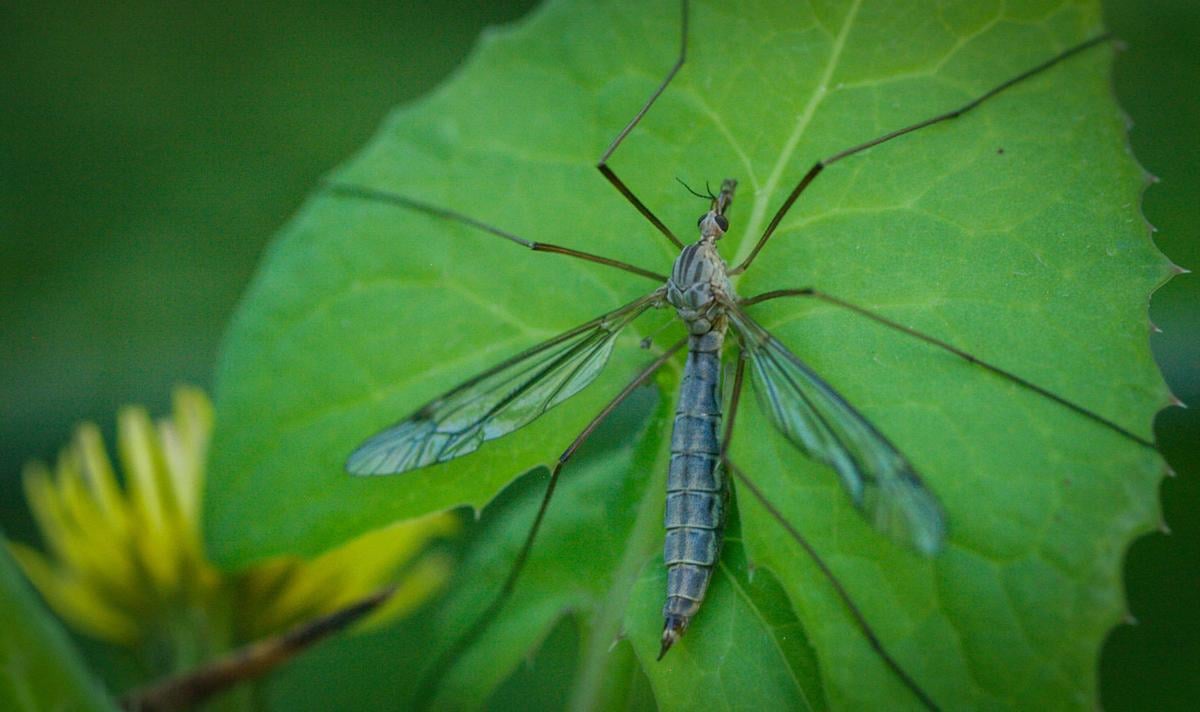The photograph is a highly detailed close-up of a dragonfly perched on a vibrant green, healthy leaf with intricate vein patterns clearly visible. The dragonfly, characterized by its six very long legs and a lengthy torso, displays transparent wings outstretched, with its bluish-greenish-gray body in sharp focus. Its black eyes are easily distinguishable. The background features an out-of-focus yellow flower located at the bottom left side, contributing to the overall natural setting, which appears to be outdoors on a cloudy day, casting subtle shadows across the scene. The dragonfly seems to be either drinking dew or feeding on the leaf’s surface, remaining very still amidst the surrounding greenery.